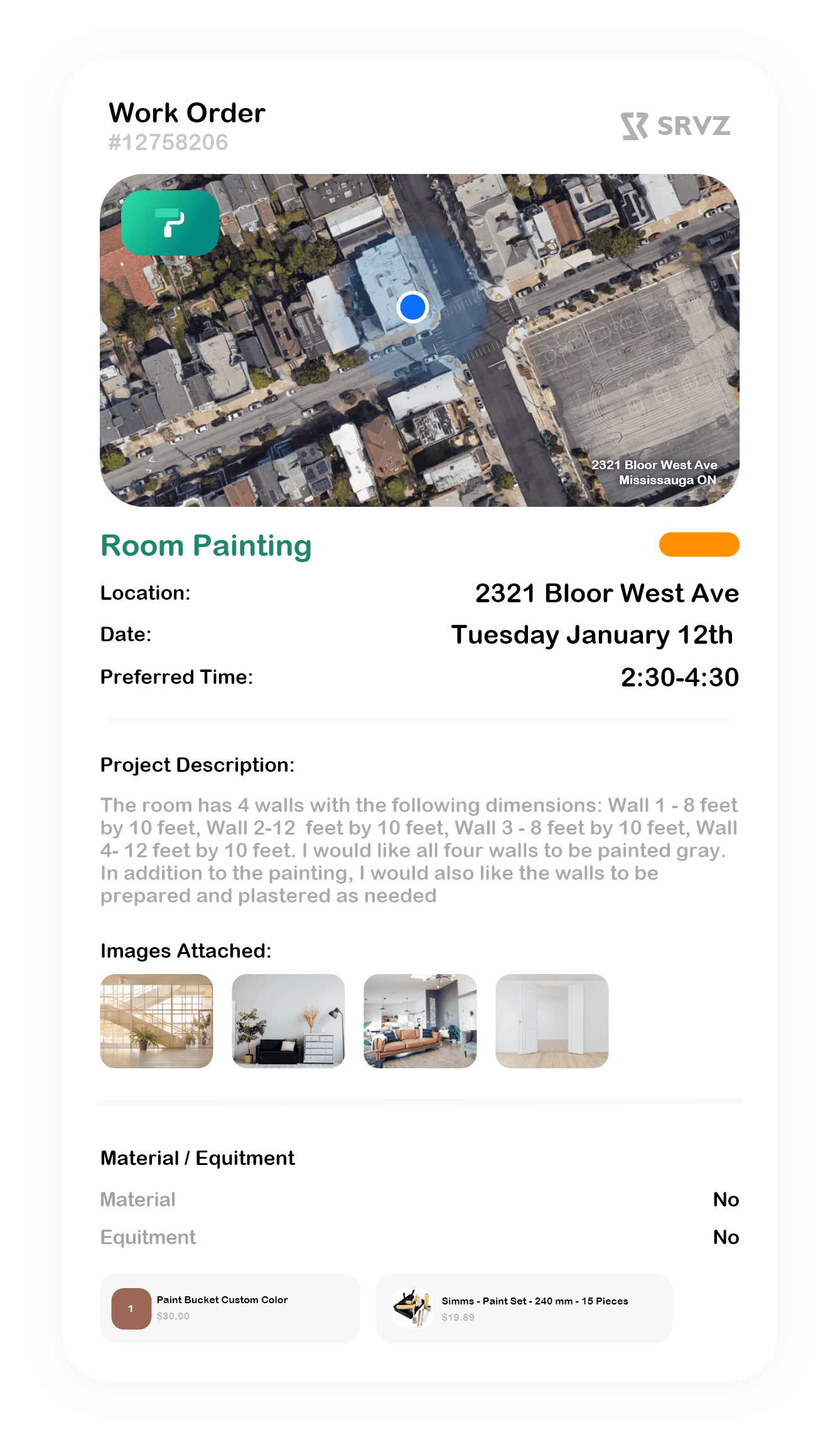This image features a work order utilizing the SRVZ system, evident from the label on the upper right-hand side. On the upper left-hand side, the document is clearly marked "Work Order" in black font, followed by the identification number #12758206. The central portion of the work order includes an aerial photograph of a street, suggesting a rural setting. 

Beneath the photograph, the document specifies the task as "Room Painting," to be carried out at 2321 Bloor West Ave. The scheduled date for the project is Tuesday, January 12th, with a preferred time slot from 2:30 PM to 4:30 PM.

The project description outlines that the room consists of four walls with specified dimensions, and all four walls are to be painted gray. Additionally, the walls require preparation and plastering as needed before painting. This detailed scope of work ensures that the necessary preparatory steps are taken for a high-quality finish.